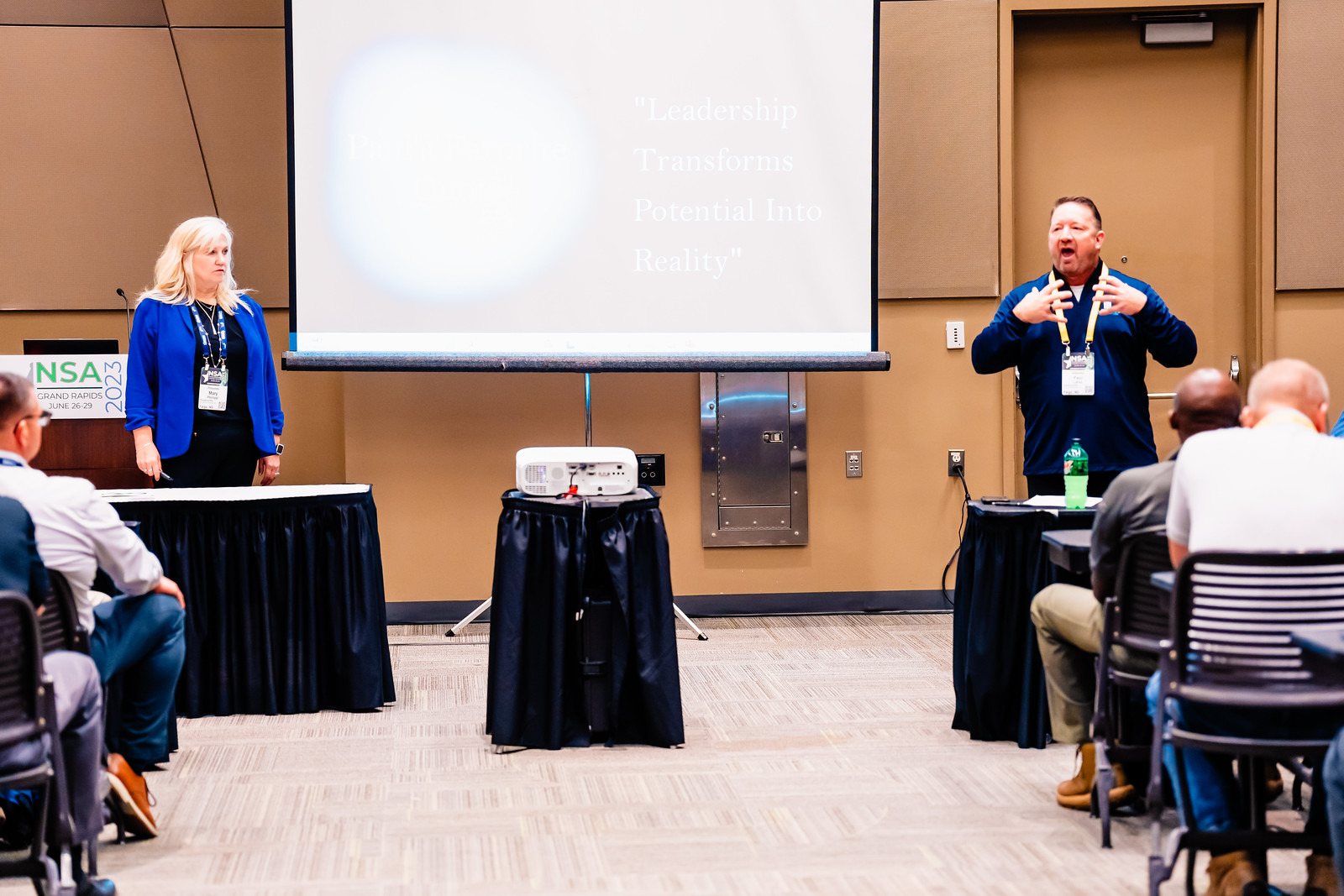In this image, a man and a woman stand at the forefront, addressing an audience seated in a large room with beige walls and a door at the back. A prominent white projection screen dominates the center, displaying a partially visible circle and indiscernible text. On the left, a blonde woman with a blue jacket and black attire, who also wears a badge, stands behind a table draped in a blue skirt. In the middle of the room, there is another small table, similarly skirted blue, holding a white projector. Standing to the right is a man dressed in a blue shirt and a lanyard, with short brown hair, a mustache, and a beard. He appears to be speaking, with his hands raised to his chest and mouth open. The room features light-colored carpeting and rows of audience members seated on either side in black chairs.